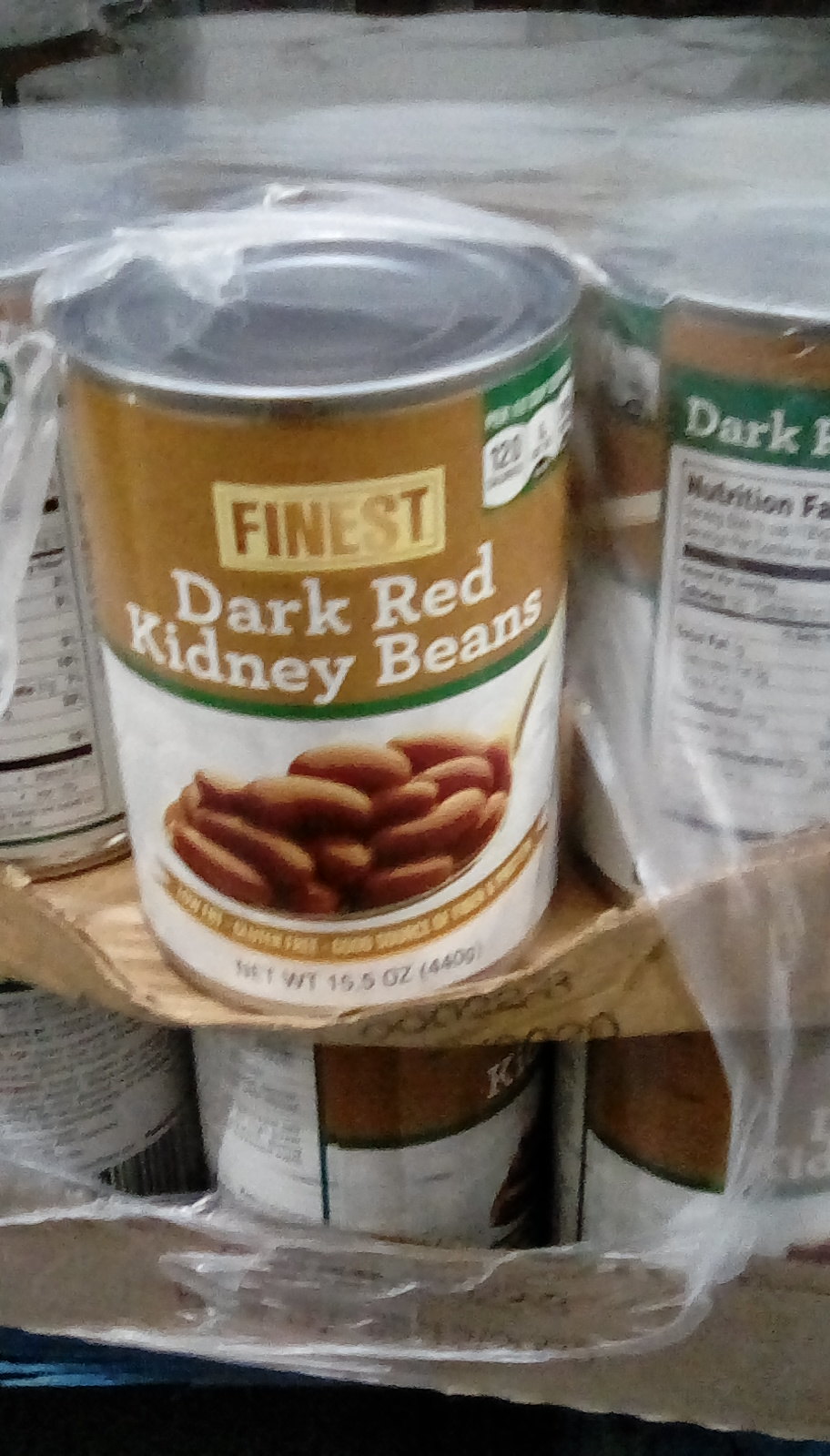The image depicts a grocery store pallet holding a shrink-wrapped case of canned dark red kidney beans. The pallet features two layers of cardboard trays stacked on top of one another. Each tray contains several cans, although the exact number is hard to determine. One can is prominently turned towards the viewer, showcasing its label in detail. The can belongs to the "Finest" brand, with a rectangular, light yellow label featuring brown lettering. The top half of the label is a lighter brown strip that reads "Finest Dark Red Kidney Beans," followed by a thin green stripe in the middle. The bottom half is mainly white, displaying a silver spoonful of kidney beans and additional details. The net weight, 15.5 ounces, is printed in black lettering at the bottom. The top right corner of the can includes a green nutritional information panel. Both cardboard cases are tightly shrink-wrapped together, indicating the beans’ high quality and the readiness for bulk purchase.